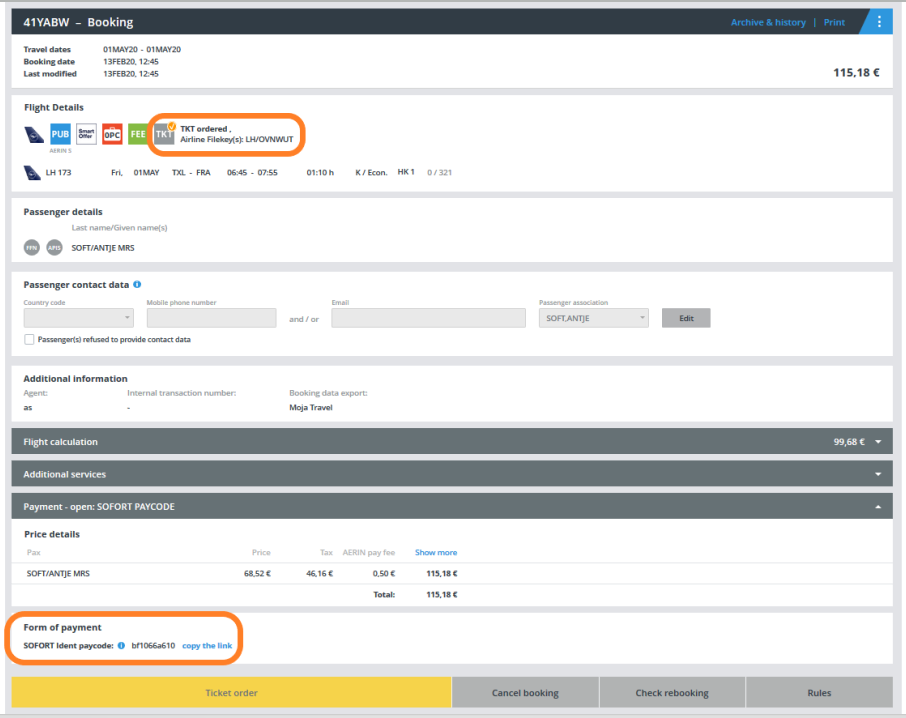The image contains various sections and information related to a booking. In the upper left-hand corner, there is a title in a gray bar that reads "41YABW - Booking." In the upper right-hand corner, there are options labeled "See Archive" and "History" along with the word "Print."

Below this, a separate section is labeled "Travel Dates," displaying May 1st. Another subsection shows the "Booking Date," which is February 13th, 2020, along with the note that it was "Last Modified" on the same date, February 13th, 2020.

The "Flight Details" section is prominently highlighted in an orange font and includes text such as "TKT Ordered" and "Airline File Keys ULH/OVNWT." Toward the bottom of the image, another circled section indicates the "Form of Payment," described as "Ident Pay Code - So Forth."